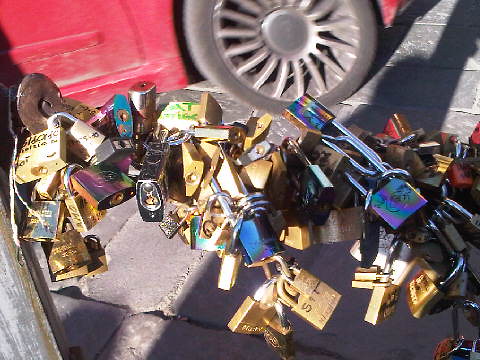This image displays a bustling collection of padlocks, commonly referred to as "locks of love," densely packed onto a horizontal bar, which appears to be part of a bike rack or similar structure. The padlocks, varying in color and design, cover the bar almost entirely and even extend onto a pillar visible on the left side of the image. There are gold, black, blue, and purple locks, with some boasting shiny patterns in blue, red, pink, and yellow. Each lock features a silver shackle, contributing to the metallic sheen of the conglomeration. One lock near the bottom has the letters "ST" inscribed in black. In the background, a red vehicle with black wheels and silver rims is partially visible, parked on a pavement made of brick concrete. The scene is reminiscent of the well-known love lock bridges, symbolizing enduring affection through the secured padlocks.